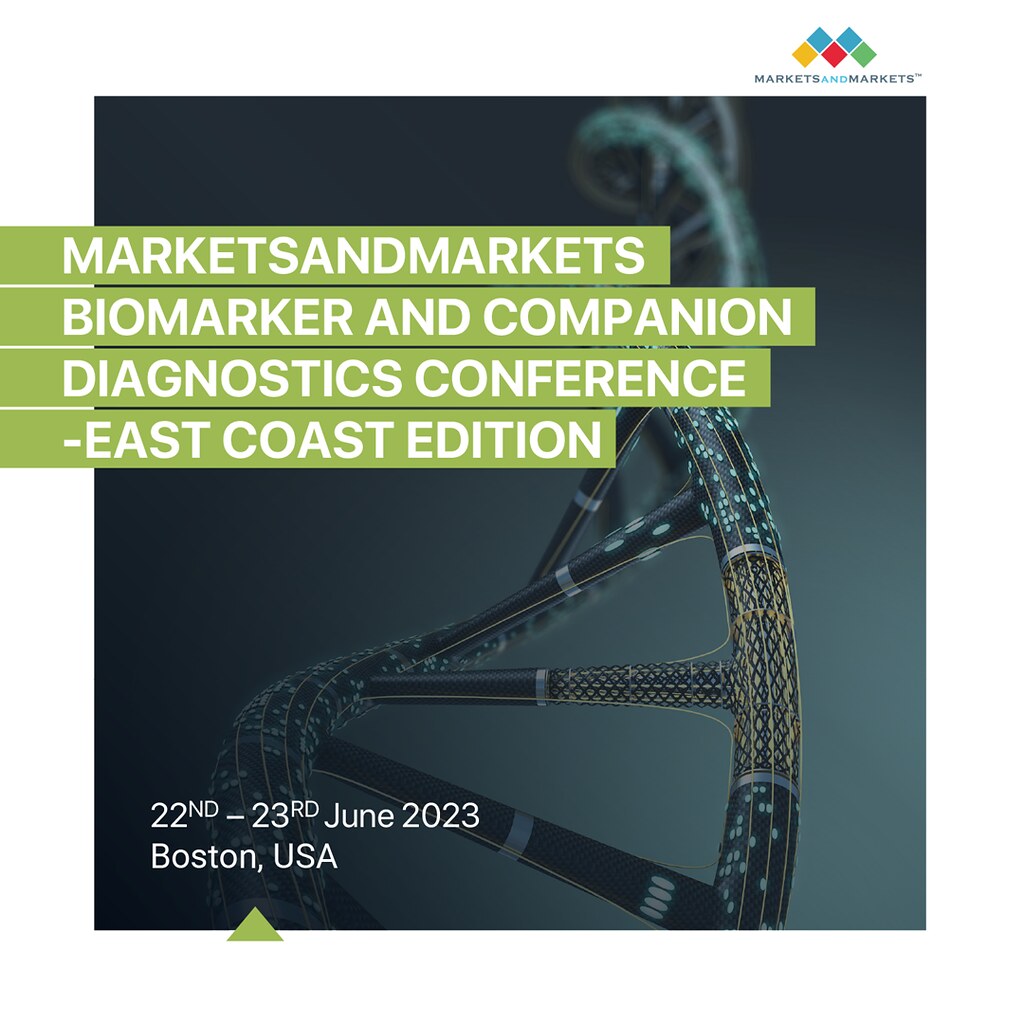This image appears to be a detailed and visually striking poster advertising the "Markets and Markets Biomarker and Companion Diagnostics Conference - East Coast Edition." The background of the poster is predominantly a dark or black color, which highlights the central 3D graphic of a coiled, DNA-like strand rendered in shades of gray and black. 

In the upper right corner, the logo is prominently displayed, consisting of five squares forming a letter "M" in blue, yellow, red, and green, alongside the text "Markets and Markets." Directly beneath this, the title of the event is clearly stated: "Markets and Markets Biomarker and Companion Diagnostics Conference - East Coast Edition." 

Additional information, including the dates "22nd to 23rd of June 2023" and the location "Boston, USA," is positioned in the lower left corner in white text, framed against the darker background. The entire image is cohesively designed to serve as a promotional piece for the conference, using a clear and consistent color scheme of black, white, blue, yellow, red, and green, which enhances the scientific and professional aesthetic of the poster.